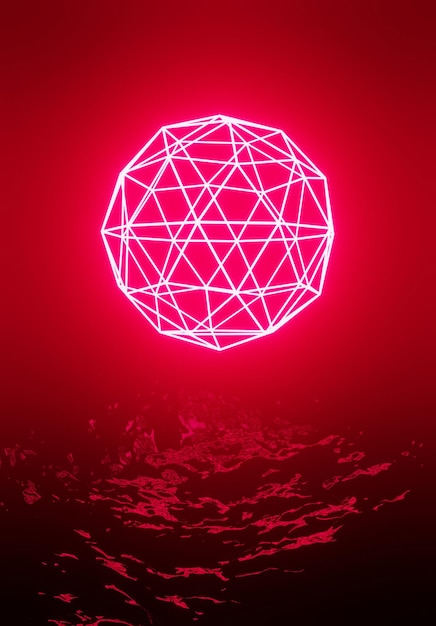The image is an abstract, AI-generated artwork with a primarily red background that transitions through varying shades, becoming darker towards the bottom. Dominating the top portion is a glowing, white-pink orb, which appears 3D and intricate, formed by thin, interwoven lines creating a spiky, geometric shape. This orb is evocative of the sun, casting a rich and bright red hue around itself. Below this central feature, the red background transforms into a textured surface with darker red and black blending, resembling waves or rugged terrain. The lower sections of the image feature splashes of red on top of darker hues, enhancing the contrast and adding to the painting's dynamic, abstract nature.